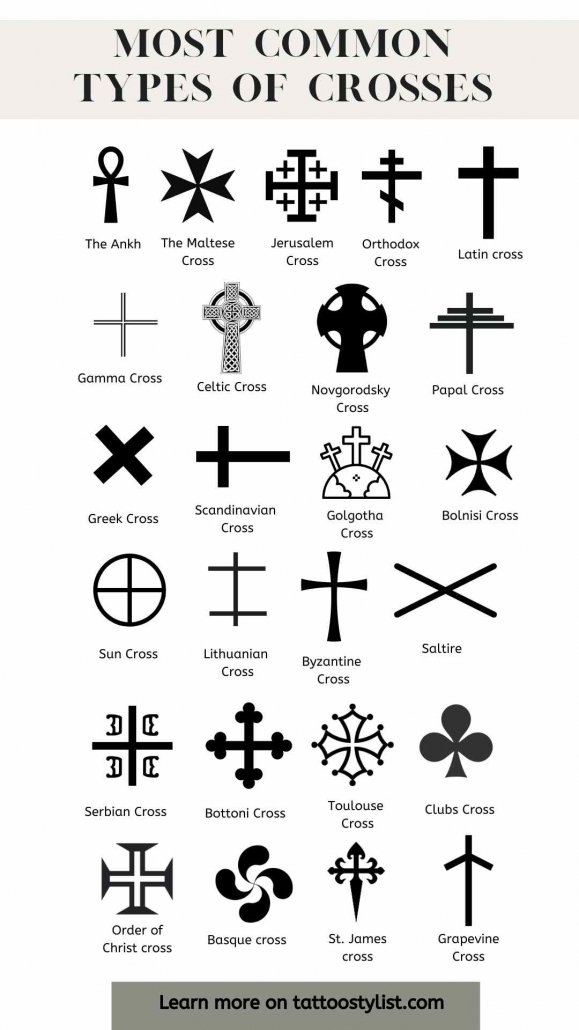This black and white image showcases a detailed array of the most common types of crosses, often used as stencils or examples for tattoo artists. The image is divided into six rows, each featuring a different cross style, meticulously drawn and labeled beneath. The list of crosses includes the Ankh, Maltese, Jerusalem, Orthodox, Latin, Gamma, Celtic, Novgorodski, Papal, Greek, Scandinavian, Golgotha, Bolsini, Sun, Lithuanian, Byzantine, Saltire, Serbian, Botony, Tall House, Clubs, Order of Christ's Cross, Basque, St. James, and Grapevine. At the top, a banner in light gray displays the black text "Most Common Types of Crosses," while a darker gray banner at the bottom reads "Learn more on tattoostylist.com." The high level of sharp detail in the stencils highlights their potential use as tattoo templates, making this image a comprehensive guide for anyone interested in cross designs.